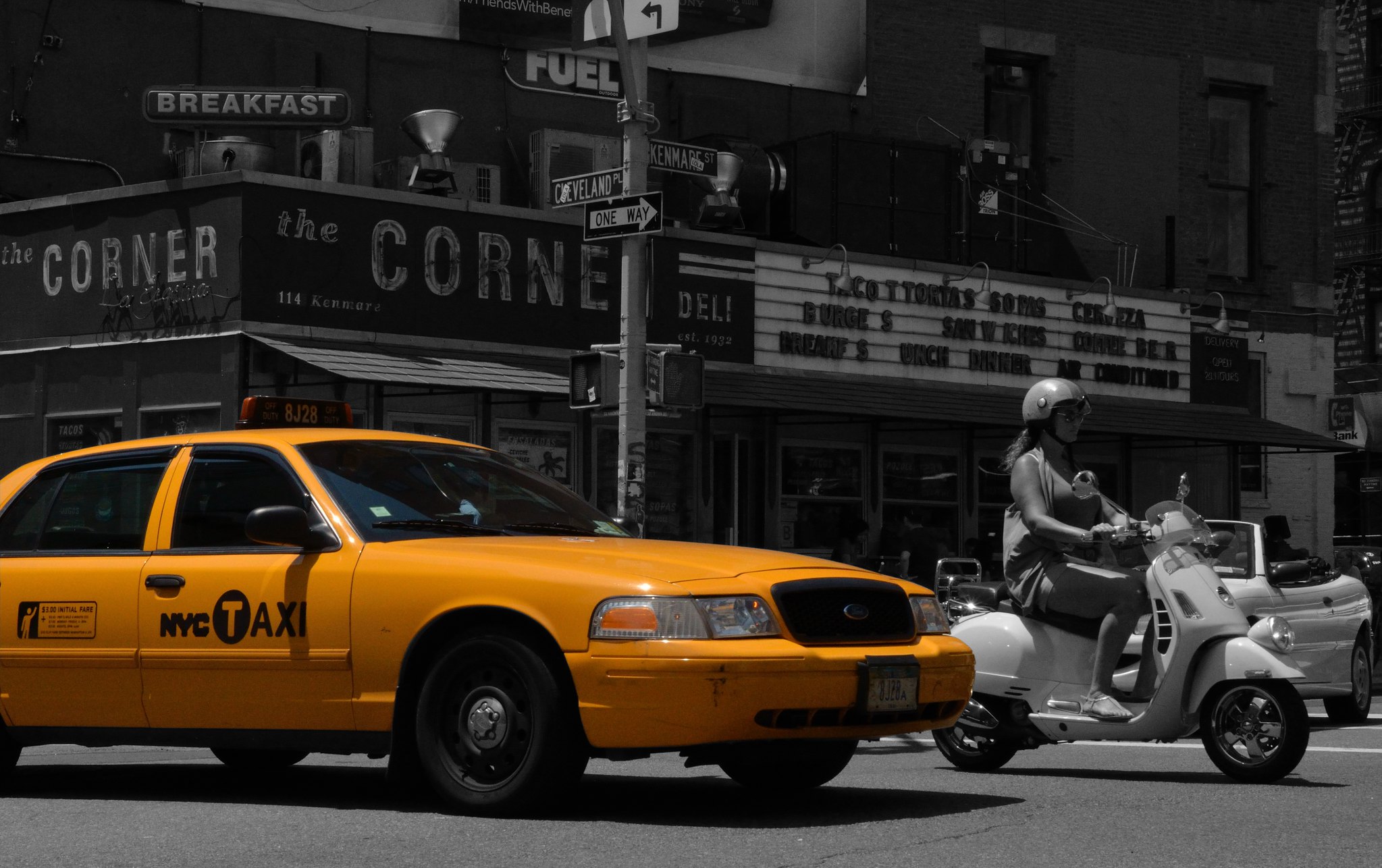In a visually striking black and white photo, color pops vividly on a single element: a yellow New York City taxi, prominently featuring black text reading "NYC Taxi" along with the identifier "8J28." The taxi is captured in motion from the left side, revealing its hood, front side, and two doors, with its black grille and tires sharply contrasting against the gray surroundings. Adjacent to the taxi, a woman clad in a shirt and shorts rides a scooter, wearing a half-helmet. In the backdrop, the streetscape is punctuated by large, imposing buildings, one of which bears the sign “The Corner,” along with smaller signs advertising breakfast, fuel, and deli options. The scene is accentuated by street signs 'Cleveland PL' and 'One Way' mounted on a substantial metal pole. A convertible car makes a turn further in the background. Additionally, a notice board with barely readable letters stands near a brick building, its windows looking down on the bustling, yet monochrome, urban tableau.